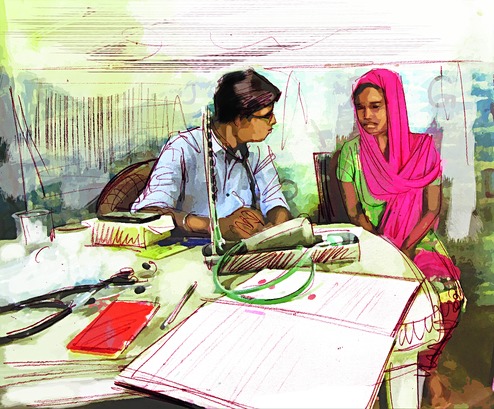The image is a vivid and colorful sketch depicting a scene involving two people. The person on the left side appears to be a doctor, identifiable by the stethoscope around his neck, glasses, and a blue long-sleeve shirt. He has brown hair and is leaning slightly towards the woman on his right, writing on a white table. The woman, who seems to be an Indian patient, is adorned in bright traditional attire, featuring a bright red or pink headscarf that drapes along her left shoulder, a neon green shirt, and a vibrantly patterned skirt composed of green, pink, and yellow hues. The two are seated in separate chairs behind a table bearing various medical instruments and items: a stethoscope, a blood pressure reader, a large open book, a patient's record, a red pamphlet-like envelope, a pen, and what appears to be a glass jar. The backdrop of the scene is a blend of blue, yellow, and green colors, contributing to the painting's lively ambiance. The overall setting is brightly lit, enhancing the clear and detailed rendering of the figures and objects in the image.